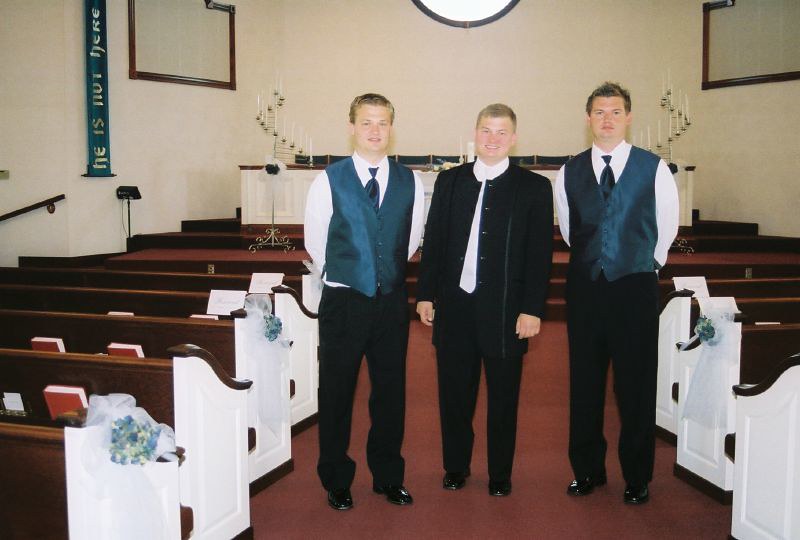The image captures a detailed scene inside a church, focusing on three men positioned at the front. The church interior has dark brown wooden pews, with white decorations draped over or painted on them, and flowers tied with white fabric present on every other pew. The floor is a reddish-brown color, and the back of each pew holds Bibles. To the left, there is a blue banner, possibly bearing a message, while candles adorn the altar area. 

Of the three men standing in the middle aisle:
- The left and right men are wearing matching white shirts, blue ties, and blue vests paired with black pants. 
- The man in the center, possibly a groom or minister, is dressed in a white shirt and a black jacket and pants, with some white accessory around his neck. 

They are presumably preparing for a wedding, given the decorative setup and their formal attire. All three men have their hands behind their backs, except the central figure, who clasps his hands in front.